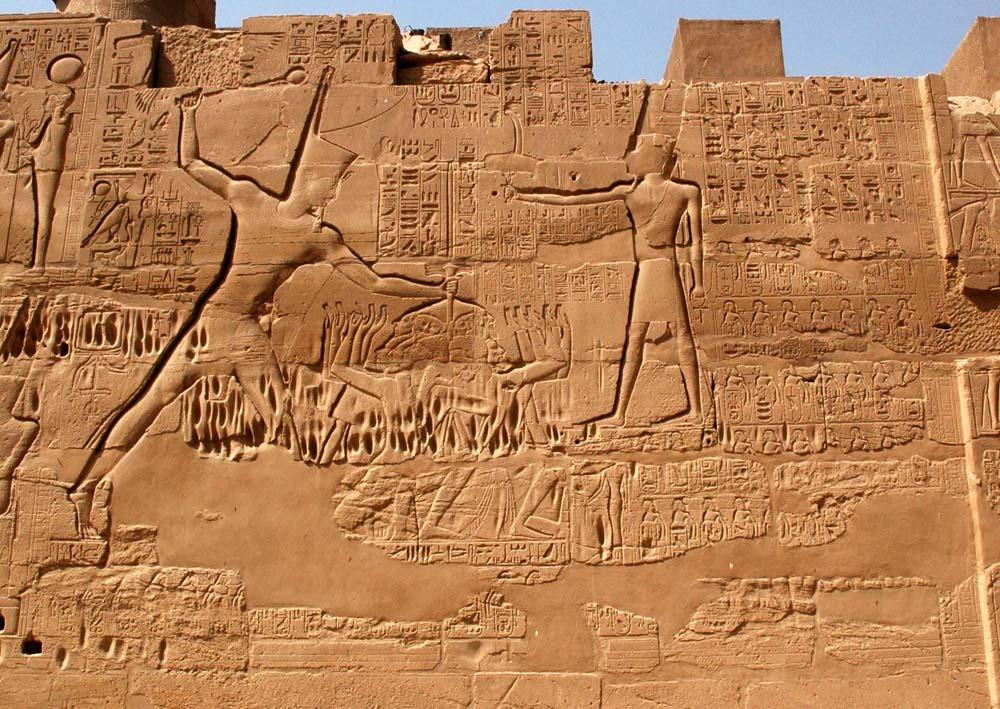The image depicts a reddish-brown wall that appears to be part of an ancient Egyptian building or potentially a fortress. The wall is adorned with detailed carvings and hieroglyphics. On the left side of the wall, there is a prominent figure, possibly a pharaoh, with his body facing forward and his head turned to the left. His left hand grips an object while his right hand is raised high, holding what looks like a rod or a weapon, as if preparing to strike. To his right, another figure stands, with his body also facing forward but his head turned to the right. This figure’s right arm is extended outward, and his left arm hangs down. Surrounding these figures are numerous other carvings and shapes, telling a rich story of ancient times. At the top of the wall, additional stone blocks and a glimpse of a pillar are visible, and the blue sky can be seen in the background, adding depth to the scene.